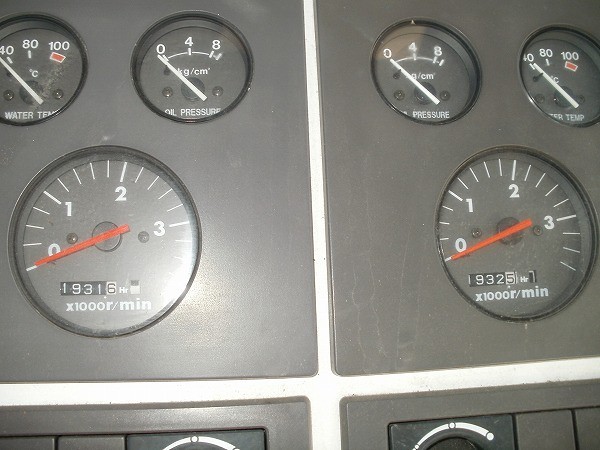The image features two adjacent panels, each equipped with three dials. The most prominent dials are located at the bottom of each panel, distinguished by their larger size. These dials are calibrated with numerals 0, 1, 2, and 3, interspersed with three tick marks between each number. Each dial has a red hand indicator and an odometer-like display at the bottom: the left panel shows a reading of 19316, while the right panel shows 19325.

Above these large dials are two smaller gauges on each panel. On the left-side panel, the upper left corner houses a dial labeled "Water Temp," marked with the numbers 40, 80, and 100. The white hand of this dial is positioned just below the number 40, indicating a relatively low temperature. Adjacent to this is another small dial labeled "Oil Pressure," marked with the numbers 0, 4, and 8. The white hand on this dial indicates just below the 0 mark, suggesting minimal oil pressure. The details and readings on the right-side panel's small dials are not specified.